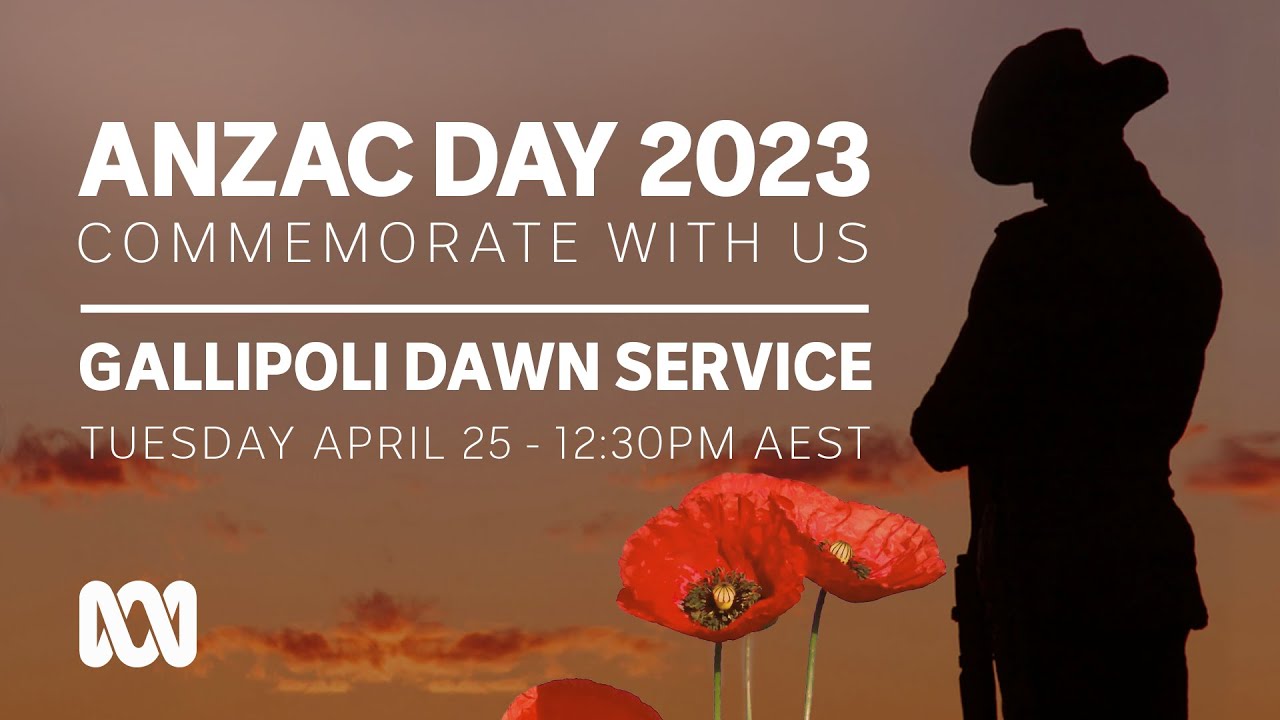In this image, we see a detailed advertisement for Anzac Day 2023. The backdrop is a nuanced brownish-gray sky, suggesting the ambiance of a sunrise or sunset, with clouds at the bottom illuminated in a striking reddish-orange hue. Dominating the right side, there's a stark black silhouette of a man, recognizable by his cowboy hat and a belt with something hanging from it. Centerpiece to the visual are green stems and red poppies, their centers a mix of burnt brown and light brown, indicating a symbolic, perhaps poignant, imagery of life and remembrance. Prominent white text overlays the center, reading "Anzac Day 2023, Commemorate with us," followed by a clean, bold line. Below this, it states "Gallipoli Dawn Service, Tuesday, April 25th, 12:30 PM AEST." A distinguishable bold logo featuring crisscrossing lines or infinity symbols anchors the bottom left corner, enhancing the solemn yet respectful tone of the announcement.